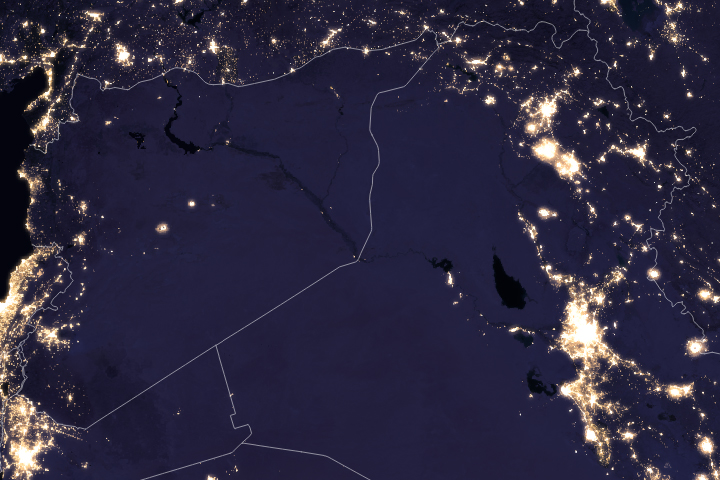The image appears to be a nighttime satellite photograph of Earth with heavily illuminated cities and towns scattered across the dark landscape. This gives the impression of various clusters of bright lights against a predominantly dark background. Adding to its complexity, the image also features white lines that resemble borders or territorial demarcations, likely indicating the divisions between countries or states. These intricate lines crisscross the image, mixing the realism of a satellite photo with the interpretive finesse of an overlay map. The scene is strikingly reminiscent of viewing space or the night sky, with the way the lights punctuate the darkness, somewhat akin to stars in the sky. Despite its abstract feel, the combination of illuminated terrains and mapped outlines suggests a deliberate attempt to blend geographical representation with illustrative details.